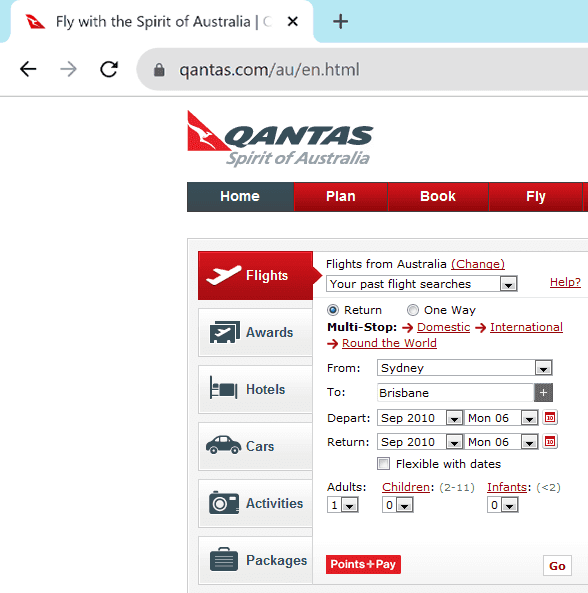A partial screenshot captured from the main Qantas website features a detailed navigation layout. At the top, a grey section resides adjacent to a white tab adorned with a distinctive red triangle enclosing a white kangaroo silhouette. Next to this emblem, the slogan "Fly with the Spirit of Australia" is prominently displayed in black, accompanied by a grey button to the right.

Further down, the background transitions to white, presenting navigation options with a black left arrow, a grey right arrow, and a black refresh icon. The web address "blacktexasisquanus.com," now greyed out, appears above another segment of white background featuring the Qantas logo: a red triangle with a kangaroo and the text "Qantas" in black below it, followed by the words "Spirit of Australia" in grey.

Below this logo, a grey button labeled "Home" in white text precedes three red buttons with white text stating "Plan," "Book," and "Fly." Continuing down the left-hand side, a vertical navigation menu lists options like "Flights" (in white text on a red background), and under a grey background, a series of categories appears in dark grey text: "Awards," "Hotels," "Cars," "Activities," and "Packages."

Included is a white box for flight searches labeled "Search from Australia." The form indicates a return flight to Brisbane dated September 10, 2010, with one adult, no children, and no infants. Though this screenshot is notably dated, it offers a glimpse into the website's functionality and design.